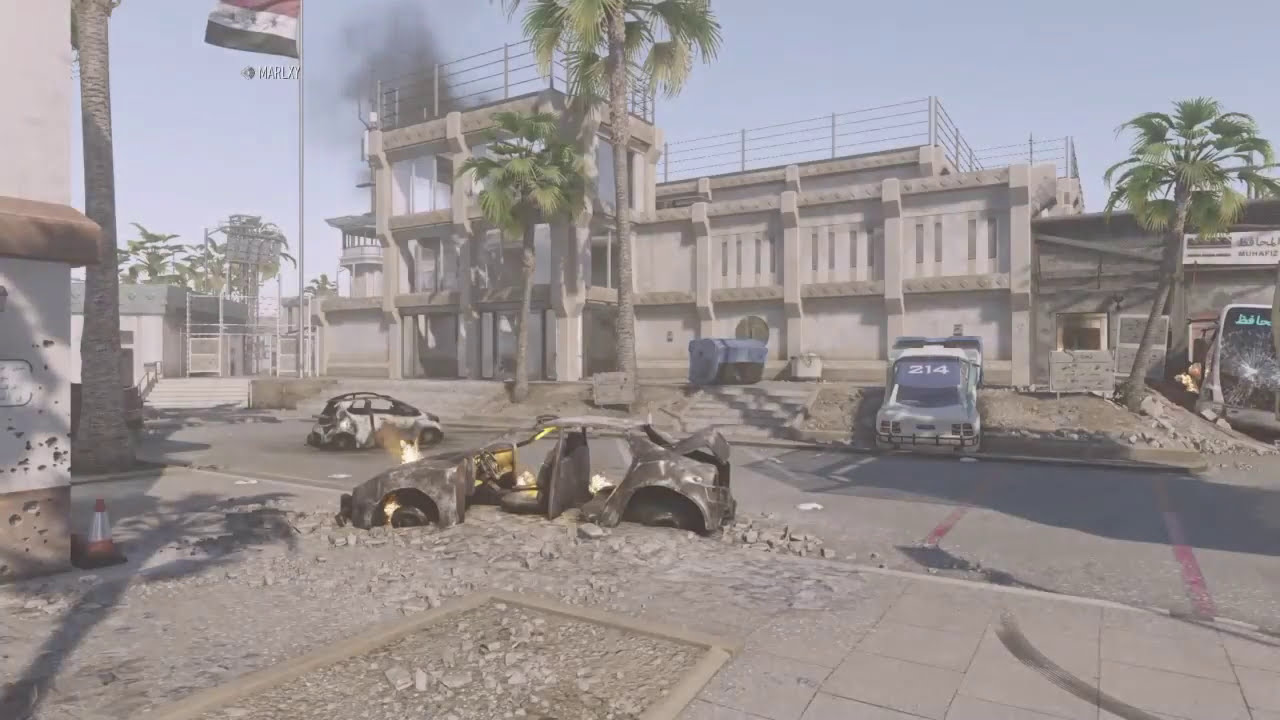This image is a clear screenshot from a video game and is horizontally rectangular, measuring roughly six inches wide by four inches tall. It depicts a devastated city street, likely in a Middle Eastern locale suggested by a prominently displayed red, white, and black flag with three black stars in its central white stripe, possibly the Syrian flag. The flagpole, situated towards the right of the scene, also features a tiny, partially readable text "M-A-R-L-X-Y" or a variation thereof in white.

The setting is outdoors with a clear blue sky, and a large, three-story, light-brown, stone building occupies the center of the composition. This building is notable for its top-level railing, suggesting an accessible walkway, and it ominously emits black smoke from its rear, indicating recent destruction possibly due to a storm or bombing. Surrounding this structure are scattered, slightly bent palm trees, contributing to the chaotic, post-disaster atmosphere.

The street itself is littered with debris and several damaged vehicles. In the foreground, a gray, four-door sports car is severely crushed, partially over the curb, and engulfed in flames. Adjacent to it is another small, white, two-door hatchback in a similar burned and damaged state, located towards the center-left. Across the street, a larger vehicle has collided with a ledge, showing relatively less damage compared to others; this might be a bus or metro with a shattered front screen. Additionally, on the far left of the image, there's a view of a building's corner, marred with bullet holes, further attesting to the violence that transpired. The street is barren, devoid of people, adding a haunting silence to the ruined urban landscape.